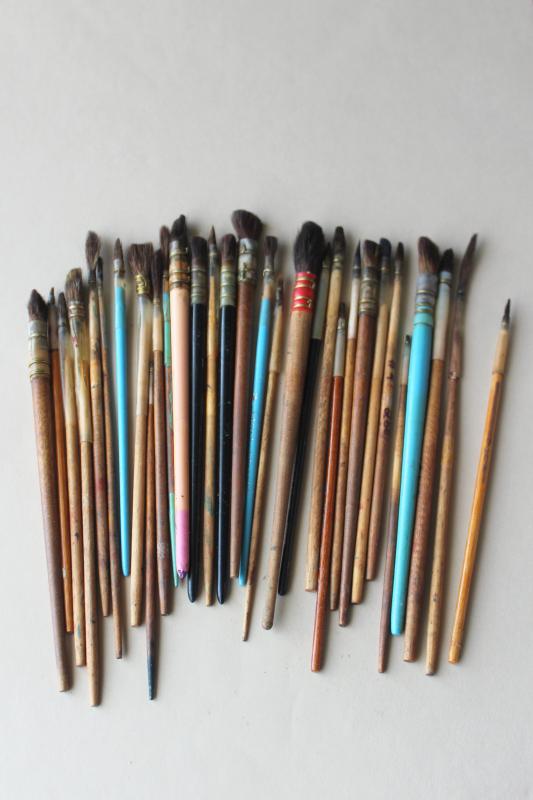The image features an assortment of around two dozen paintbrushes of varying sizes and colors, set against a white or gray backdrop. These paintbrushes are haphazardly arranged, with some handles sticking out at the top and bottom. The brushes appear well-used and well-loved, exhibiting signs of wear and remnants of paint. Most of the handles are wooden, painted in hues of light blue, dark blue, peach, and pink, with a rustic-looking furrow securing the bristles. Among the collection, a few brushes bear Japanese or Chinese kanji, suggesting they may be sumi brushes typically used for traditional Japanese or Chinese calligraphy and painting. The bristles vary in thickness and density, hinting at their use in diverse artistic techniques.